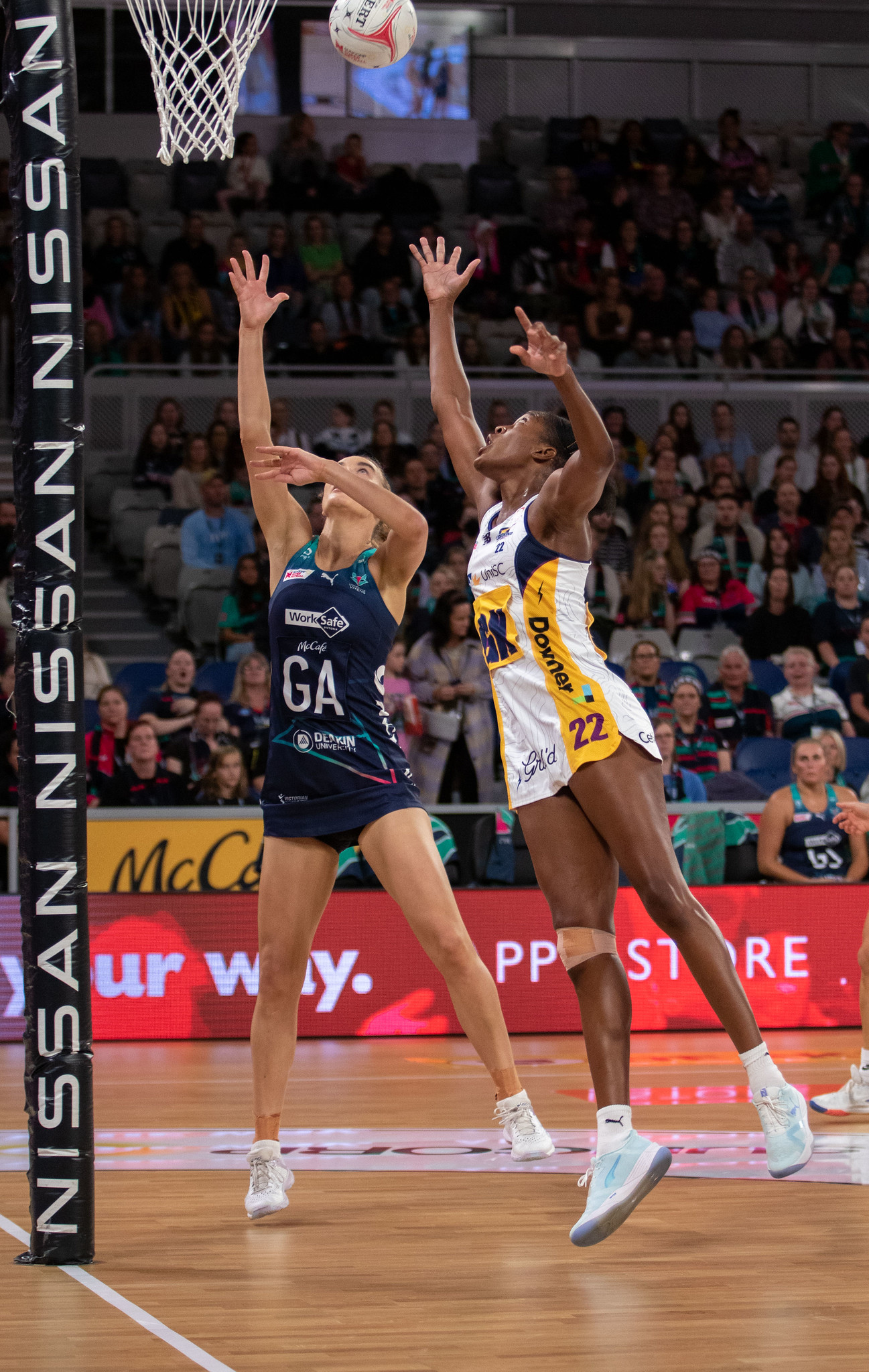The image captures an intense moment during a women's collegiate basketball game. Two players are positioned under a basketball goal, reaching up towards a white basketball that's been shot from off the side of the frame. The player on the left, wearing a dark blue uniform with "GA" emblazoned on it, is a white woman. On the right, an African American woman wears a white uniform with gold stripes and a knee wrap on her right leg. Both players have their arms extended and legs straightened as they leap towards the ball. The basketball goal features a black pole with "Nissan, Nissan, Nissan" printed in white lettering along its protective foam pad. 

In the background, a packed stadium full of spectators watches intently. The image offers a close-up of the action, highlighting the physical effort and determination as both athletes compete for possession of the ball. The overall setting is vividly captured, with the dynamics of the game and enthusiastic crowd forming an essential backdrop to this moment on the court.